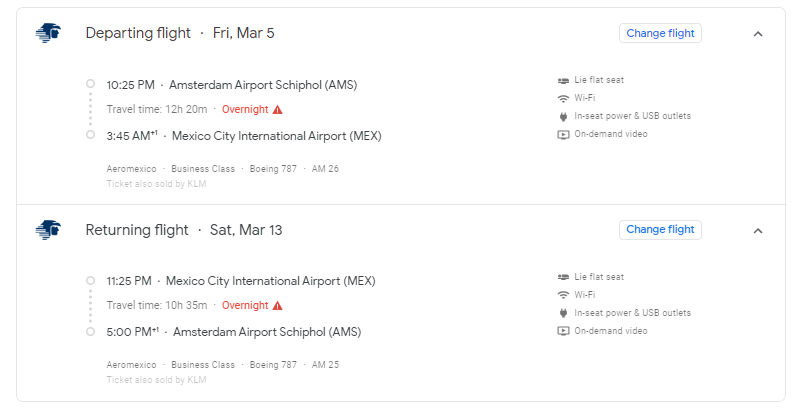The image contains two rectangular boxes detailing flight information. The top box illustrates a departing flight scheduled for Friday, March 5th at 10:25 p.m. from Amsterdam Airport Schiphol (AMS). The travel time is 12 hours and 20 minutes, with the flight arriving overnight at 3:45 a.m. in Mexico City International Airport (MEX). This flight is operated by Aeromexico in business class on a Boeing 787 aircraft, flight number AM 26, and tickets are also sold by KLM. On the right side of this box, there is a button labeled "Change Flight." Beneath it, the amenities include a lie-flat seat, Wi-Fi, in-seat power and USB outlets, and on-demand video.

The bottom box details the return flight scheduled for Saturday, March 13th at 11:25 p.m. from Mexico City International Airport (MEX). This flight has a travel time of 10 hours and 35 minutes, arriving at 5:00 p.m. the following day at Amsterdam Airport Schiphol (AMS). Again, the flight is operated by Aeromexico in business class on a Boeing 787 aircraft, flight number AM 25, with tickets also available through KLM. Amenities for this flight include a lie-flat seat, Wi-Fi, in-seat power and USB outlets.